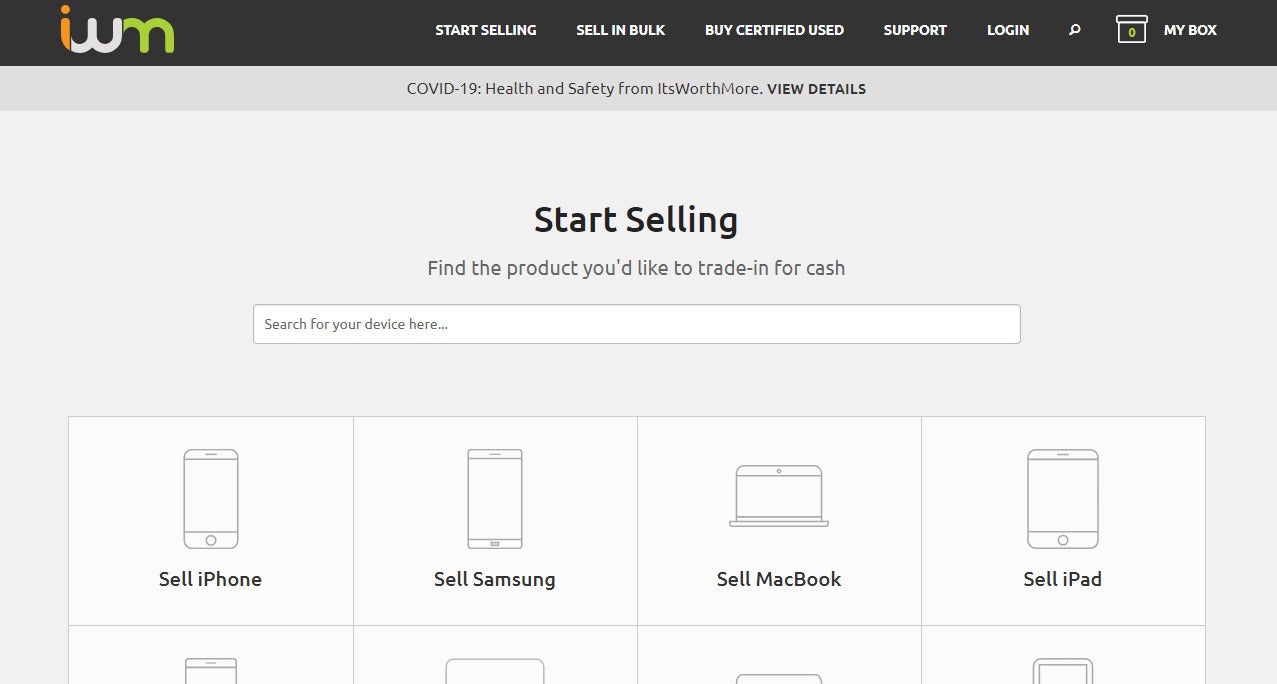The image displays a webpage with a structured layout and a corporate aesthetic. At the very top, a narrow, dark gray or black border spans the width of the page. Directly beneath this is a slightly lighter gray border, giving the top section a distinct, layered appearance. The main background of the page is an even lighter shade of gray.

In the black top banner on the left is the IWM logo, where 'I' is orange, 'W' is white, and 'M' is green, hinting at a corporate branding or logo. To the right of the logo, there is a navigation menu with several options: "Start Selling," "Sell in Bulk," "Buy Certified Used," "Support," and "Log In." A search icon is also present, along with a box showing zero items, likely representing a checkout cart, and another labeled "My Box."

Below this dark banner is a lighter gray banner at the top of the page featuring a health and safety notice regarding COVID-19 from It's Worth More, with "View details" possibly being a hyperlink due to its bold print.

Continuing downward, the main body of the page begins with a prompt to "Start Selling." It instructs users to "Find the product you'd like to trade in for cash," accompanied by a search bar for product searches. Below this, several categorized panels are displayed, including options to "Sell iPhone," "Sell Samsung," "Sell MacBook," and "Sell iPad." The page shows the beginning of another row of panels, although content below this point is cut off in the image.